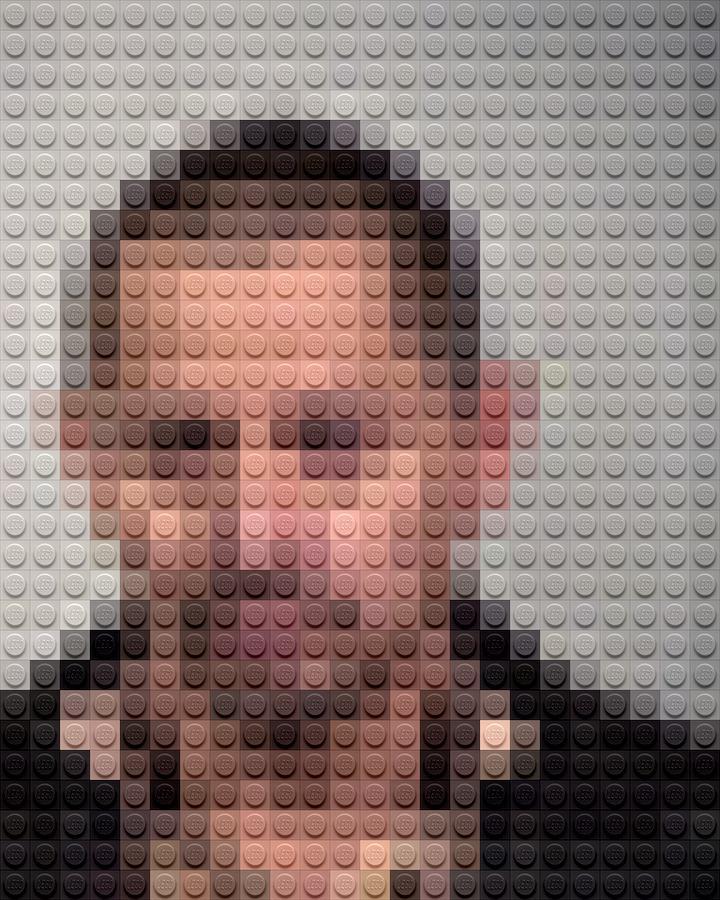This detailed color photograph, featuring a portrait of a white man with short dark hair, showcases an innovative use of Lego pieces to create a lifelike image. The subject, who might have a hint of a mustache and beard stubble, appears to be wearing a black jacket or shirt. Set against a light gray background, the man's face is positioned towards the bottom left, facing the viewer. The image, in portrait orientation, utilizes various Lego pieces in shades of skin color, brown, black, pink, white, and gray to meticulously craft his features. The special filter applied gives the portrait an abstract, impressionistic quality with a texture reminiscent of a rubber mat with a round coin pebble finish, adding depth and a unique illustrative technique to the composition.